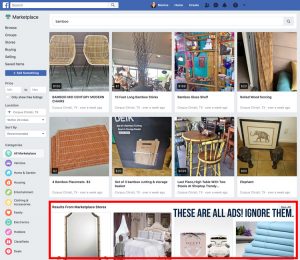This image is a screenshot from Facebook Marketplace, characterized by the signature blue border of the platform at the top. On the left side, there is a long, white rectangular search box. Due to the small size of the image, the text is unreadable, but we can identify a left sidebar in a light grayish-blue color with the word "Marketplace" at the top, followed by an unreadable list of options.

Below the search box, there are additional white search fields, each accompanied by unreadable text. The main section of the screenshot displays two rows of photos, with four images in each row. 

In the top left corner, there is a photo of two brown plastic chairs. On the second row, one image features a wooden chair beside a small, round wooden table. At the bottom, a red rectangular border highlights a message written in blue capital letters: "THESE ARE ALL ADS!" followed by the instruction to "IGNORE THEM."

Among the four images within the red rectangle, the lower right corner depicts what appears to be a stack of light blue towels. The left image shows a tall mirror, similar to those typically attached to bedroom dressers.